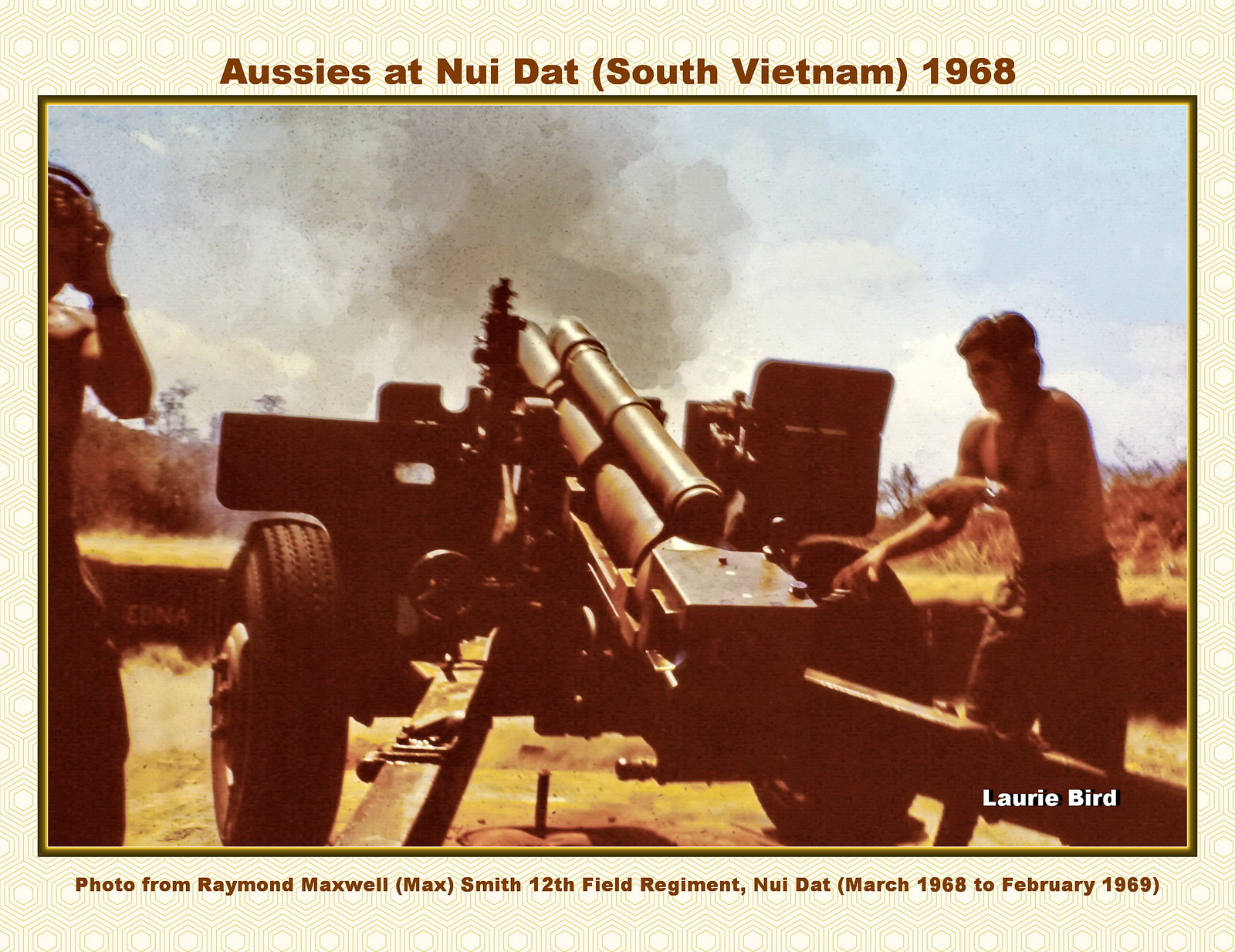This detailed photograph, taken by Lori Byrne in 1968, captures a striking moment during the Vietnam War. The scene features two shirtless Australian soldiers from the 12th Field Regiment at Nui Dat, South Vietnam, as they stand behind a massive, two-wheeled military artillery cannon amid a backdrop of a blue sky. The men are visibly bracing themselves, covering their ears against the deafening roar of the cannon they have just fired, evidenced by the thick, gray smoke billowing into the air. The picture, with its earthy tones of dirt and sand, and the contrasting greens and browns of the artillery and surroundings, also carries a historical caption in brown text at the top: "Aussies at Nui Dat, South Vietnam, 1968." Below the image, another inscription reads, "Photo from Raymond Maxwell and Max Smith, 12th Field Regiment, Nui Dat, March 1968 to February 1969." This evocative image offers a poignant glimpse into the raw intensity of wartime operations.